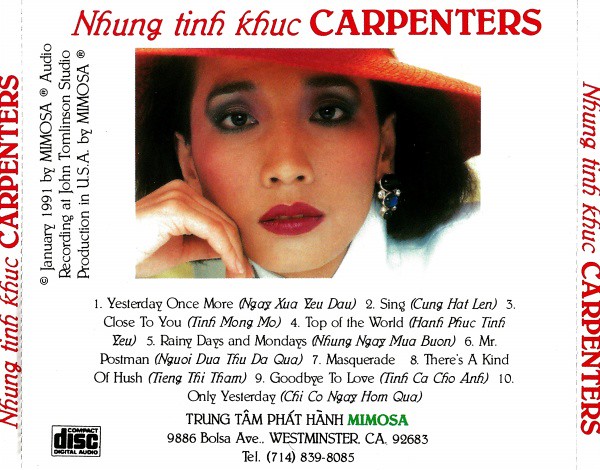The cover of this music CD features a clean, minimalist design with textual and visual elements set against a white background. At the top of the cover, bold, uppercase text spells out "NHUNG TINH KHÚC" with the English word "Carpenters" directly beneath it. Below this title, a picture of a woman occupies the middle section. The woman is seen from her upper shoulders to near the top of her head, adorned in a striking red sun hat and matching red lipstick. She has bluish eyeshadow and wears earrings with blue gems. Her outfit includes a white shirt with a tall collar, adding a touch of elegance.

The woman’s right arm is positioned leaning against her face, creating a casual yet sophisticated pose. Below her image, a black lettered text lists song titles which include: 
1. Yesterday Once More
2. (They Long to Be) Close to You
3. Top of the World
4. Rainy Days and Mondays
5. Please Mr. Postman
6. This Masquerade
7. There’s a Kind of Hush
8. Goodbye to Love
9. Only Yesterday

Further down, an address is given: "9886 Bolsa Avenue, Westminster, California, 92683," along with a contact telephone number "714-839-8085".